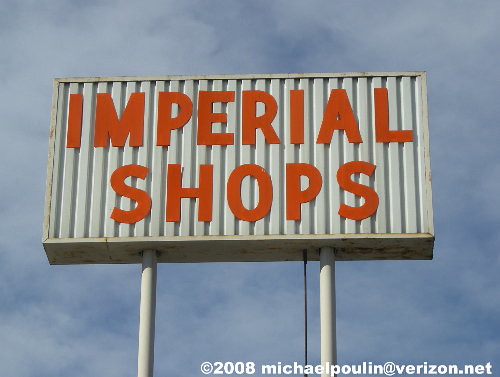This photograph showcases a tall store sign mounted on two round white metal poles, positioned high in the sky. The sign itself is a rectangular white metal board displaying the words "IMPERIAL SHOPS" in large, prominent orange capital letters. A black cord is visible running along the left side of the right pole. Below the sign, in small white text, it reads "© 2008 Michael Poulin, P-O-U-L-I-N, at Verizon.net." The background features a blue sky with a gentle haze of white clouds, providing a serene backdrop.